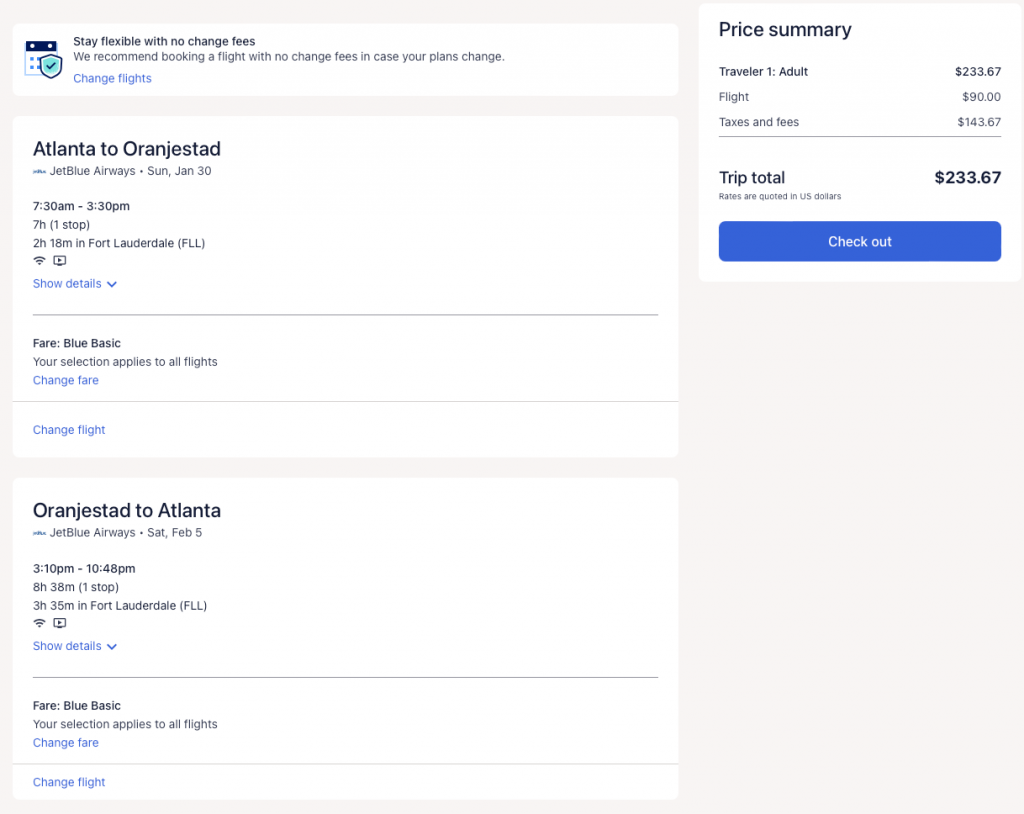A screenshot of a JetBlue flight booking checkout page is displayed. The left side of the page details the flight itinerary. The outbound flight is from Atlanta to Oranjestad, scheduled to depart on Sunday, January 30th, with a departure time of 7:30 AM and an arrival time of 3:30 PM. The return flight from Oranjestad to Atlanta is set for Saturday, February 5th. 

On the right side of the page, a price summary is presented. It outlines the cost for one adult traveler. The flight fare is $90, while the taxes and fees total $143.67, bringing the trip's grand total to $233.67. Below the price summary, there is a blue rectangular button with the word "Checkout" in white text, offering the user the option to finalize their purchase.